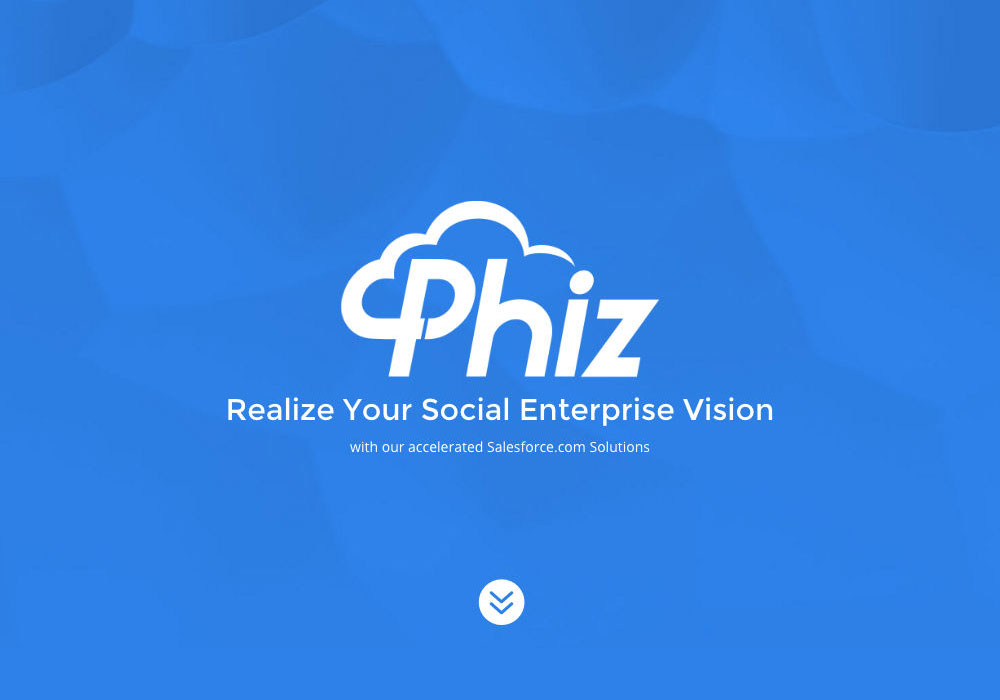The image is a blue, slightly graduated card, resembling a crumpled piece of paper that has been laid flat. At the center of the card, there is a white logo for "PHIZ," spelled P-H-I-Z. The design incorporates a cloud flowing from the top of the 'P' and arching over the letters. Below the logo, the text reads, "Realize your social enterprise vision with our accelerated Salesforce.com solutions." At the very bottom of the card, there is a round white circle featuring two downward-pointing arrows, suggesting it can be clicked to navigate to the next page. This card appears to be an advertisement or a business card for a company offering specialized Salesforce.com solutions.